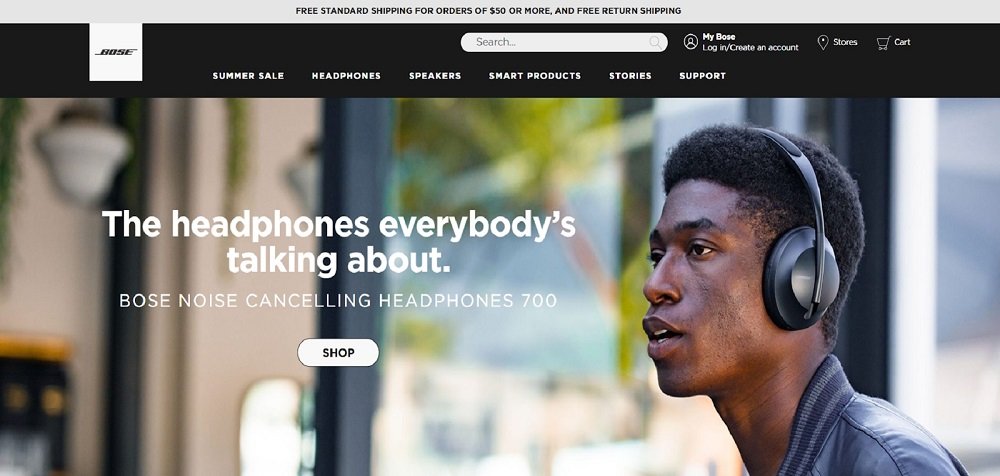The promotional image features a meticulous layout with a light gray border at the top, displaying the text "Free standard shipping for orders of $50 or more and free return shipping" in black. Directly beneath this is a black band housing a white square logo of "BOSE" in uppercase letters. 

Below the logo, a navigation menu is presented with options for "Summer Sale," "Headphones," "Speakers," "Smart Products," "Stories," and "Support." A search bar is positioned above with options for "My BOSE," "Login," and "Create an Account." Accompanying icons include a pinpoint symbol labeled "Stores" and a shopping cart symbol labeled "Cart."

The main background is slightly blurry, depicting elements such as a light fixture, a window, a tree, and possibly a shelf or bookcase. Dominantly displayed in white text is the phrase, "The headphone everybody's talking about," followed by "BOSE Noise Cancelling Headphones 700" in smaller capital letters. Below this text, there's a white oblong button with the word "Shop" in black capital letters.

On the right side of the image is a sharply dressed Black man with a box-style haircut, adorned with the featured BOSE Noise Cancelling Headphones 700 and wearing a dark-colored jacket, adding a touch of human connection to the promotional material.